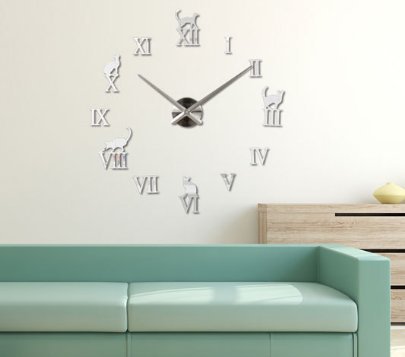This photograph features a modern, minimalist living room with a stylish flair. Dominating the scene is a large, eye-catching clock that may have been digitally added to the image. This clock, with its steel-grey face and Roman numerals, commands attention, occupying roughly 25% of the photograph. The clock shows the time as 10:10 and is adorned with the whimsical silhouettes of cats, one perched atop each key number: 12, 3, 6, 8, and 10. 

The living room itself includes a light teal, almost seafoam-colored couch or chaise lounge, contributing to the room's modern aesthetic. Behind the couch, a very light, almost bleached-out wooden dresser adds to the minimalist decor. Atop the dresser sits a small, flattened vase. The background is completed with an off-white, beige-toned wall, providing a neutral canvas that enhances the clock's striking design and the overall sophisticated atmosphere.